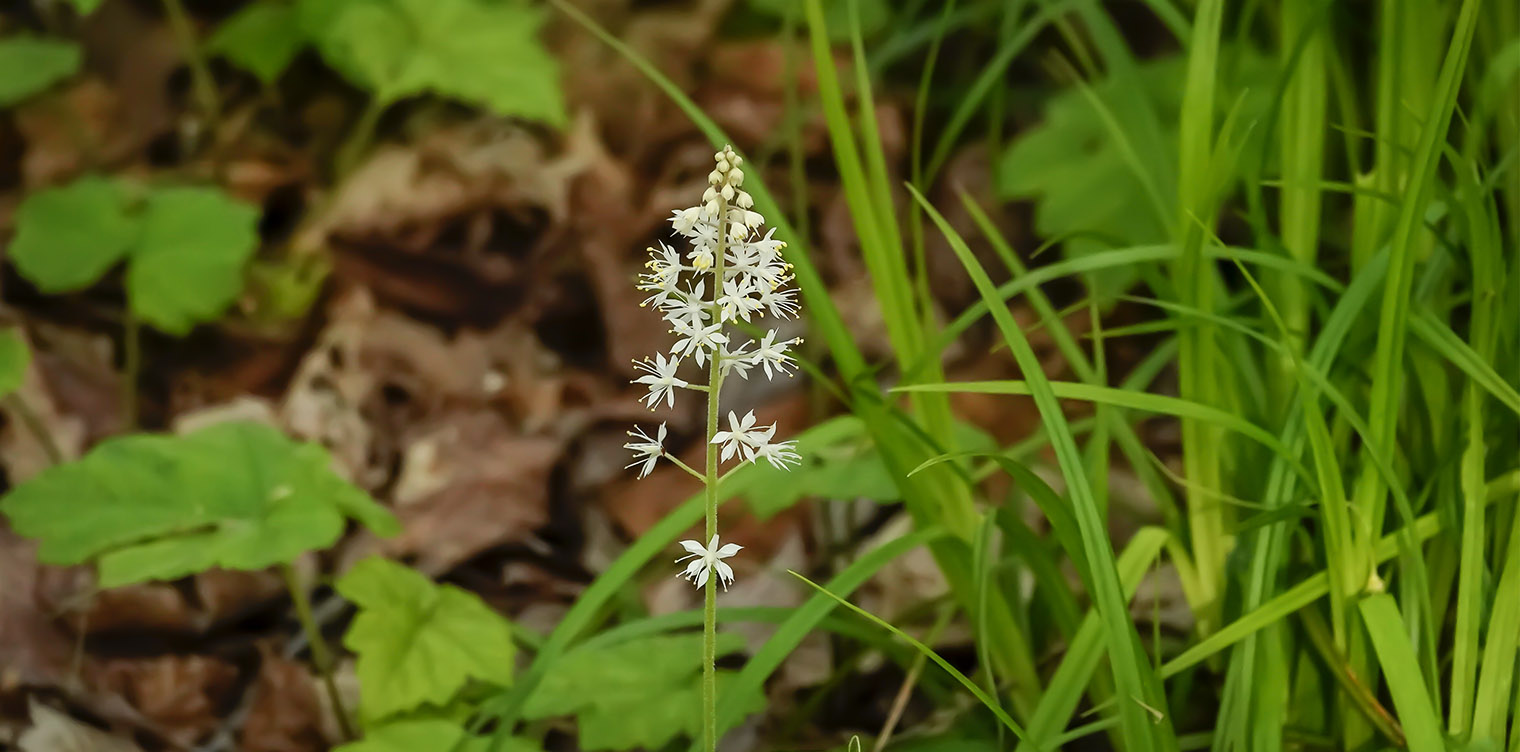In this detailed outdoor photograph, a lone, slender white flower dominates the center. Emerging from a green stalk, it isn't fully bloomed, showcasing a dozen or so tiny buds. These white buds and small flowers taper off toward the top, with subtle hints of yellow peeking through. The background features a tapestry of plants, blurred into different shades of green and brown. The right side foreground is teeming with bright green grass and long strands that rise above the flower, contrasted by the taller fronds and leaves scattered on the left. Brown, dried leaves intermix on the far left, painting a faint autumnal backdrop. This delicate interplay of greenery and dried foliage frames the modest yet captivating white flower at the heart of the image.